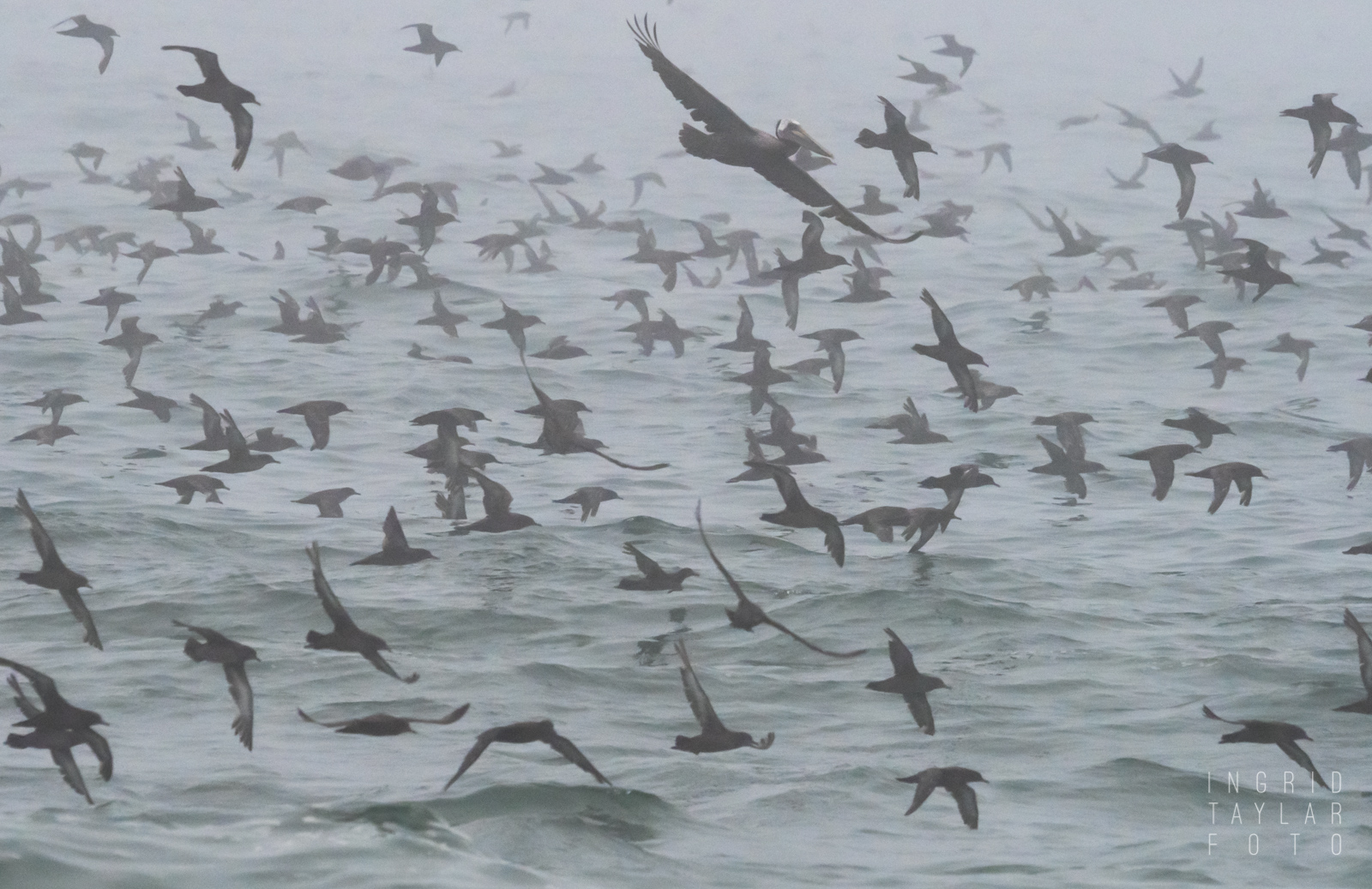In a captivating black and white photo by Ingrid Taylor, a vast swarm of black birds fills the misty, fog-shrouded sky over a choppy body of water, likely an ocean. The scene is painted in varying shades of gray, giving it an older, timeless feel. The water below, distinguished by faint waves and a blend of darker gray to light green hues, serves as the backdrop for the mesmerizing avian dance. Birds are depicted in multiple stages of flight, their wings either outstretched or pointed downwards, creating a dynamic and swirling movement throughout the image. In the crowded composition, at least fifty to a hundred birds can be seen occupying the foreground, midground, and background, with some even swooping low to touch the water's surface. Of these, one prominent bird with a large wingspan and a noticeable white beak stands out at the top middle, its form striking against the sea of dark feathers, adding a specific focal point to this ethereal, atmospheric capture.